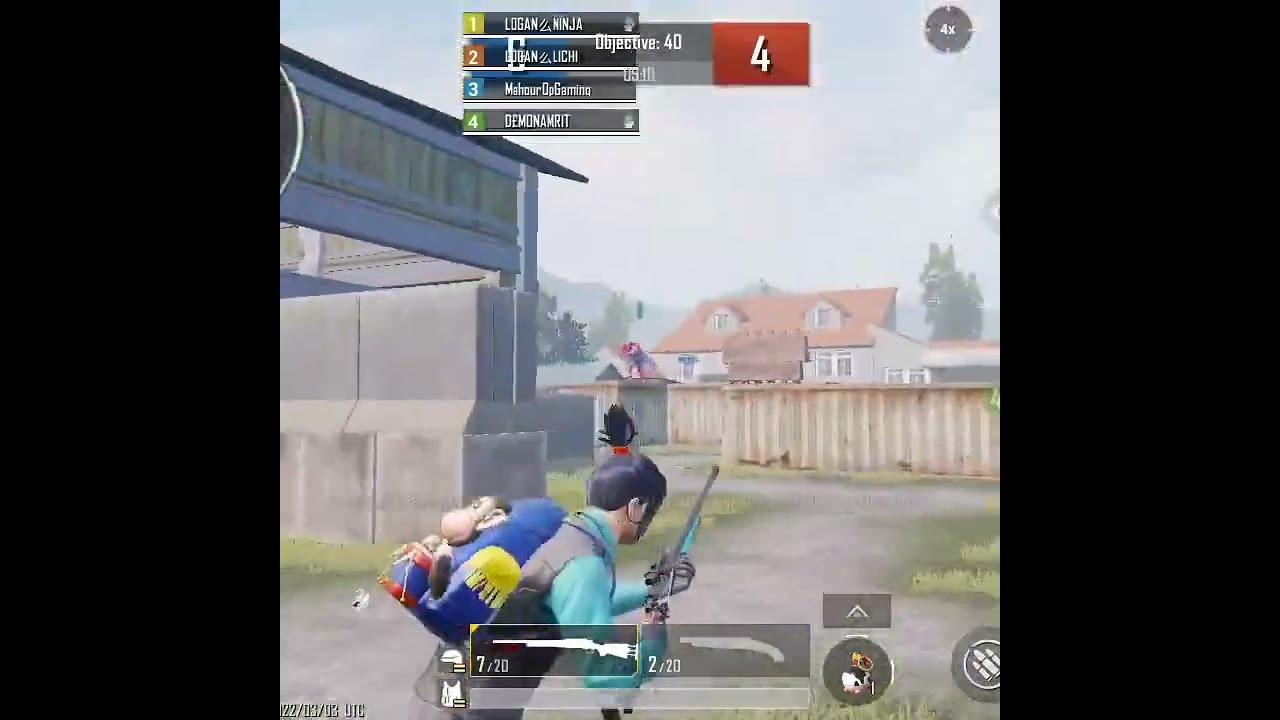The image is a detailed screenshot from a video game featuring a character viewed from behind. The character, an Asian man with black hair tied into a high ponytail held by a dark orange circle, is dressed in teal clothing on his arms and a gray vest. He is equipped with a rifle that has a black barrel and a teal stock, and on his back is a distinctive blue backpack adorned with a yellow section resembling shoulders and a monkey sticking out from it.

In the game's user interface, the upper section lists four player names in vertical alignment: Logan Ninja, an obscured second name listed with 'Object 40' beside it, Mahur de Gaming, and Demaret. There is a gray circle with a white interior in the bottom right corner, displaying an emblem of three bullets. The sides of the screenshot feature black bars about an inch and a half wide.

The backdrop of the scene includes a hazy sky and a house with a clay arched roof and a yellow wall with light brown vertical strips. Flanking the house are green trees, while a gray pathway bordered by green grass leads up to the structure. The overall graphic quality suggests a lower resolution or older video game.